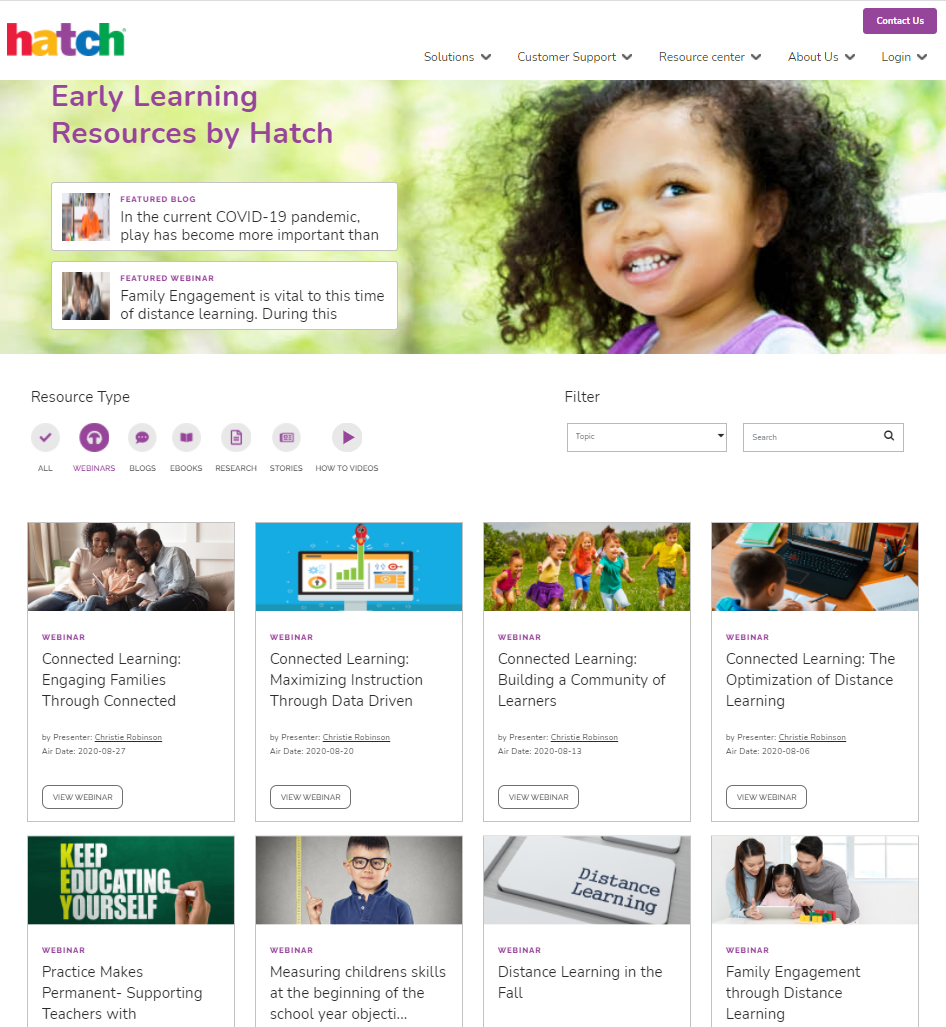The image is a screenshot of the Hatch website. The Hatch logo is prominently displayed in the top left corner, showcasing vibrant, multicolored letters: the H is red, the A is yellow, the T is purple, the C is blue, and the second H is green. To the right of the logo, the navigation menu includes clickable options for "Solutions," "Customer Support," "Resource Center," "About Us," and "Login," each accompanied by a downward arrow indicating more information is available.

In the top right corner, there is a standout purple button with white text that says "Contact Us." Just below the header, the main image features a joyful toddler, a young Black girl smiling and looking up to her right. The girl is set against a blurred, green background suggestive of a woodland area. To the left of her, in purple text, the page reads "Early Learning Resources by Hatch."

Beneath this section, a black button offers further options, though the text is partially cut off. It reads: "Featured Blog: In the current COVID-19 pandemic, play has become more important than..." and "Featured Webinar: Family Engagement is vital to this time of distance learning during this..."

The left sidebar lists various resource types for users to explore, including "All Webinars," "Blogs," "E-books," "Research Stories," and "How-To Videos." The section is currently focused on webinars, indicating users can filter by topic or search on the right side of the screen. The listed webinar topics include:
- Connected Learning: Engaging Families Through Connected Learning
- Connected Learning: Maximizing Instruction Through Data-Driven Strategies
- Connected Learning: Building a Community of Learners
- Connected Learning: The Optimization of Distance Learning
- Practice Makes Permanent: Supporting Teachers
- Measuring Children's Skills at the Beginning of the School Year
- Distance Learning in the Fall
- Family Engagement Through Distance Learning